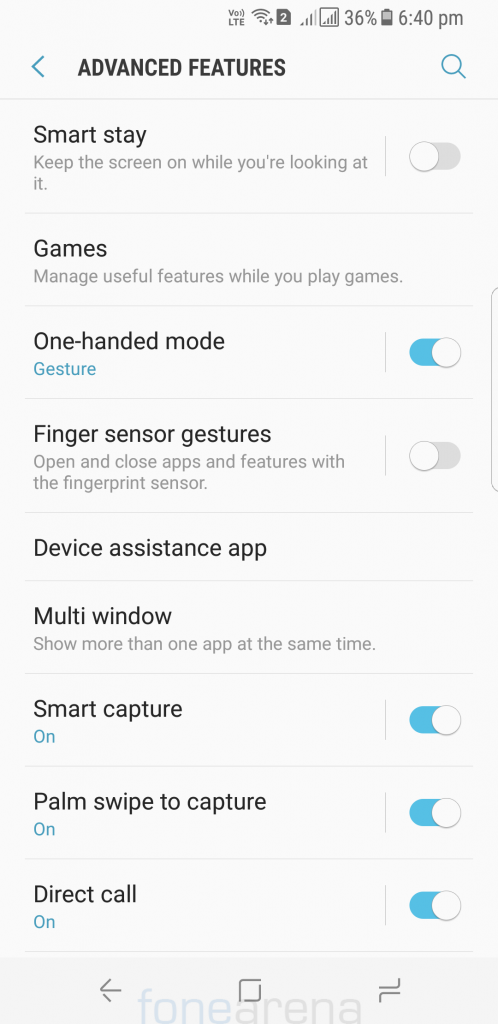A screenshot of an Android phone's settings menu, specifically the "Advanced Features" section. The screenshot lists several functionality options, each with a toggle switch on the right side to enable or disable them. The available features include:

1. **Smart Stay**: Keeps the screen on while the user is looking at it.
2. **Games**: Manages useful features during gameplay.
3. **One-Handed Mode**: Enables easier use of the phone with one hand.
4. **Finger Sensor Gestures**: Allows opening and closing of apps and features using the fingerprint sensor.
5. **Device Assistant App**: Settings related to the default assistant app.
6. **Multi Window**: Allows the display of more than one app at the same time.
7. **Smart Capture**: Captures screenshots with additional options.
8. **Palm Swipe to Capture**: Allows the user to capture screenshots by swiping the screen with their palm.
9. **Direct Call**: Enables dialing a contact by bringing the phone to the ear.

In this user's settings, the toggles indicate that "One-Handed Mode", "Smart Capture", "Palm Swipe to Capture", and "Direct Call" are enabled, while "Smart Stay" and "Finger Sensor Gestures" are disabled. The layout and design of the interface confirm it is an Android device, as it significantly differs from the settings interface on Apple devices.